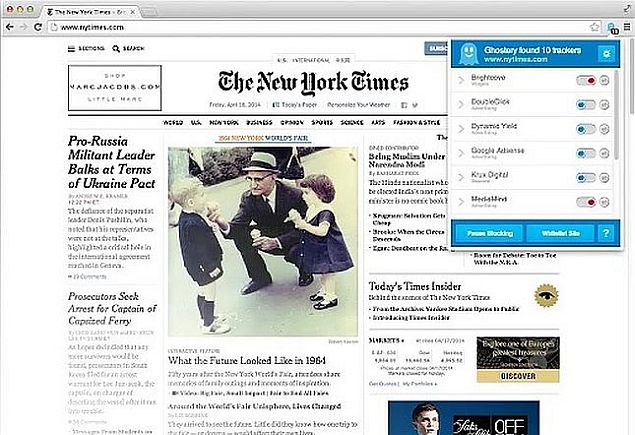Screenshot of the New York Times website taken on a MacBook with an older Mac OS. The website has a white background with a gray top bar containing the close, minimize, and maximize window buttons. The address bar is white and displays "www.nytimes.com." On the right side of this bar, there's a highlighted extensions button showing information about website trackers, specifically an extension named "Ghost Boy" which has identified 10 trackers. Beneath this, there are options toggled on or off.

In the main area of the screenshot, the New York Times website is open, featuring an image of a man crouching with two children standing in front of him. Several headlines are visible, including "Pro-Russia Militant Leader Backs Terms of Ukraine Pact" and "What the Future Looked Like in 1984."